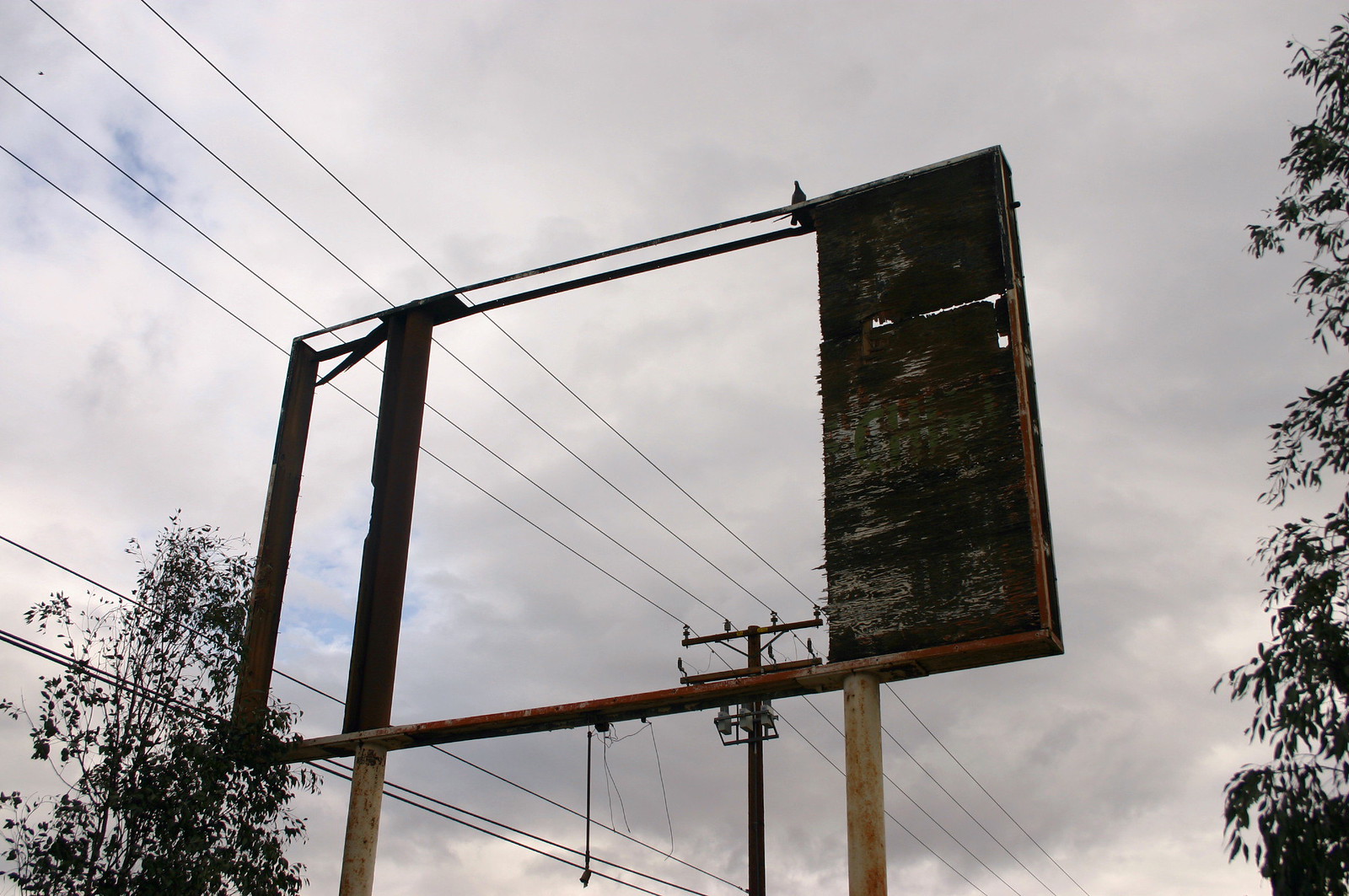This color photograph captures a poignant scene set against a predominantly cloudy sky, with patches of blue breaking through. Dominating the center of the image is a dilapidated, rectangular billboard frame, missing most of its original structure. The billboard stands as a mere shell of its former self, with only remnants of wooden planks clinging to the right side, now worn and frayed. Perched gracefully on the top right of the billboard is the silhouetted figure of a bird. Thin black power lines intersect the image horizontally from a pole arising from the center, adding an element of stark contrast against the sky. In the background, the landscape is complemented by the tops of trees peeking in from the lower left and right corners, creating a sense of depth and framing the desolate yet compelling scene.